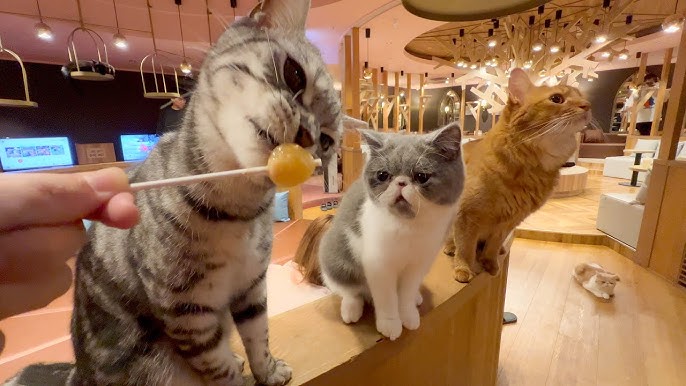In this vibrant and cozy interior, reminiscent of a cat cafe, we see a lively scene featuring five cats and intricate details for feline enjoyment. Central to the image is a kitchen island hosting three cats. On the left is a white, black, and gray cat with stripes along its limbs, curiously sniffing or licking a yellow lollipop held by a person. Next to it, a gray and white cat intently watches the lollipop. On the far right, an older orange cat gazes off into the distance as if contemplating a leap from the counter.

Beyond the counter, the room is well-lit with hanging lights and adorned with wooden decor, giving off a warm and inviting atmosphere. There are several sofas—a white one on the right side and a brown one towards the back. The flooring is a light pine wood, adding to the airy feel. In the background, there are more cats, including an orange and white cat on the floor to the right, and a black cat hanging from a gold structure in the top left. TVs are also visible, enhancing the social environment where people and cats intermingle.